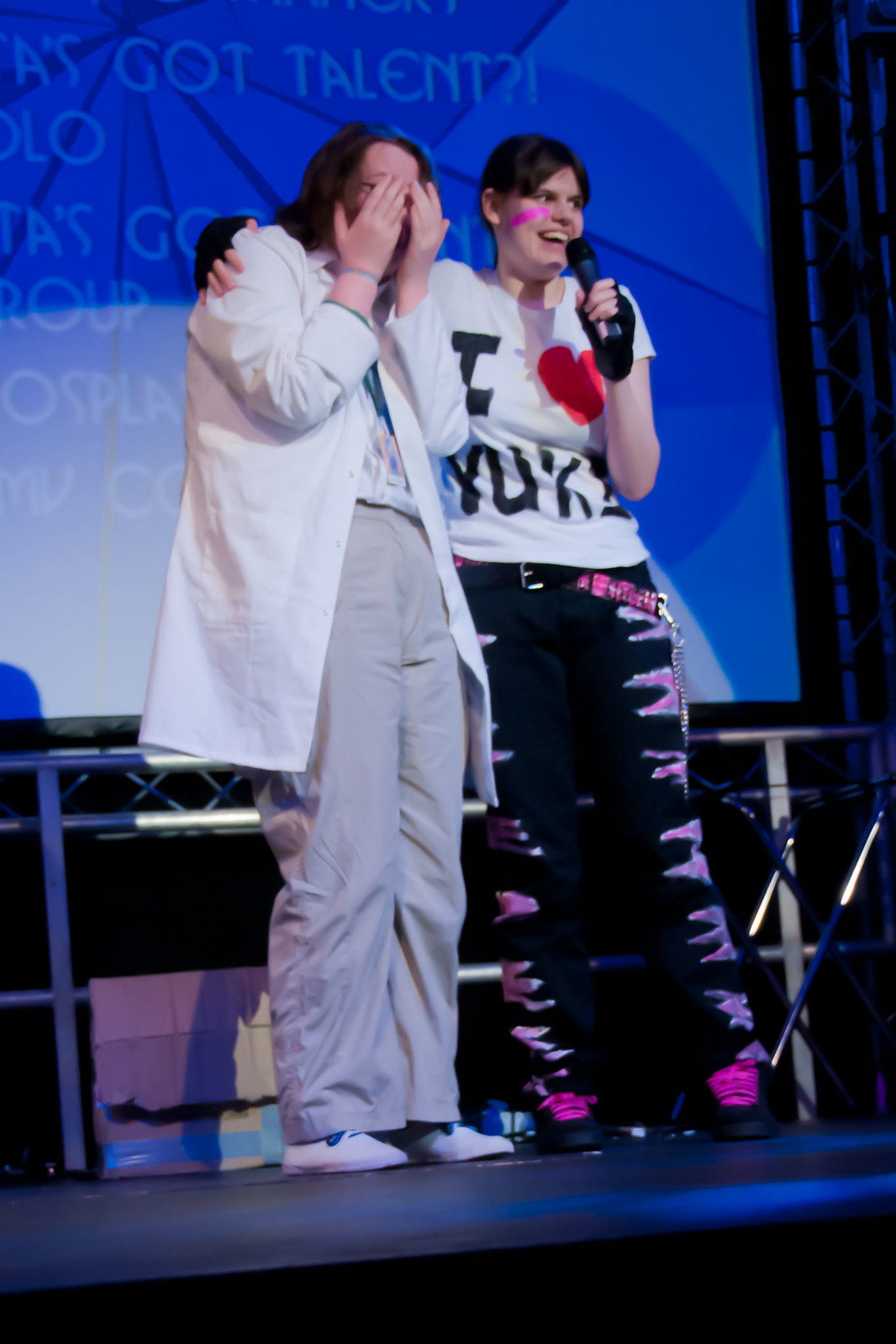The image captures two women on a stage, centrally positioned in front of a large, partially legible screen that seems to display text reminiscent of "Got Talent," suggesting a possible talent show setting. The stage is dimly lit, with various colors including black, gray, white, pink, blue, and purple accentuating the scene. 

The woman on the right is prominently holding a microphone in her left hand, wearing a white t-shirt emblazoned with "I ♥ Y-U-K-E" or similar lettering. Her outfit is notable for its black jeans adorned with pink embellishments, black shoes with pink shoelaces, and dark fingerless gloves. She also has a blue stripe painted on her cheek and wears a big smile, suggesting she's engaged in a lively performance or speech.

To her left, the second woman is covering her face with her hands, possibly out of embarrassment. She wears a white coat, khaki pants, and white shoes. Both women have brown hair. The background features a screen with a blue kaleidoscopic design, further contributing to the vibrant and dynamic atmosphere of the venue.